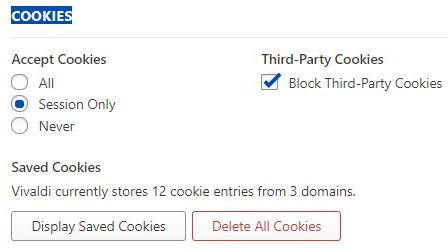The image showcases a cookie management page within the Vivaldi browser. At the top, the title "Cookies" is prominently highlighted in dark blue. The interface is divided into two main sections: "Accept Cookies" and "Third-Party Cookies." 

On the left, under "Accept Cookies," there are options to manage cookie preferences:
- "All"
- "Session Only"
- "Never"

To the right, under "Third-Party Cookies," there is an option to block these cookies, indicating that the user has chosen to block third-party cookies for this session. 

Below these sections, "Saved Cookies" details that the browser currently stores 12 cookie entries from three domains. Two buttons are available:
- "Display Saved Cookies" in plain black text
- "Delete All Cookies" in a light lavender color

Overall, the page is designed to be simple and user-friendly, allowing easy navigation and selection of cookie management preferences.